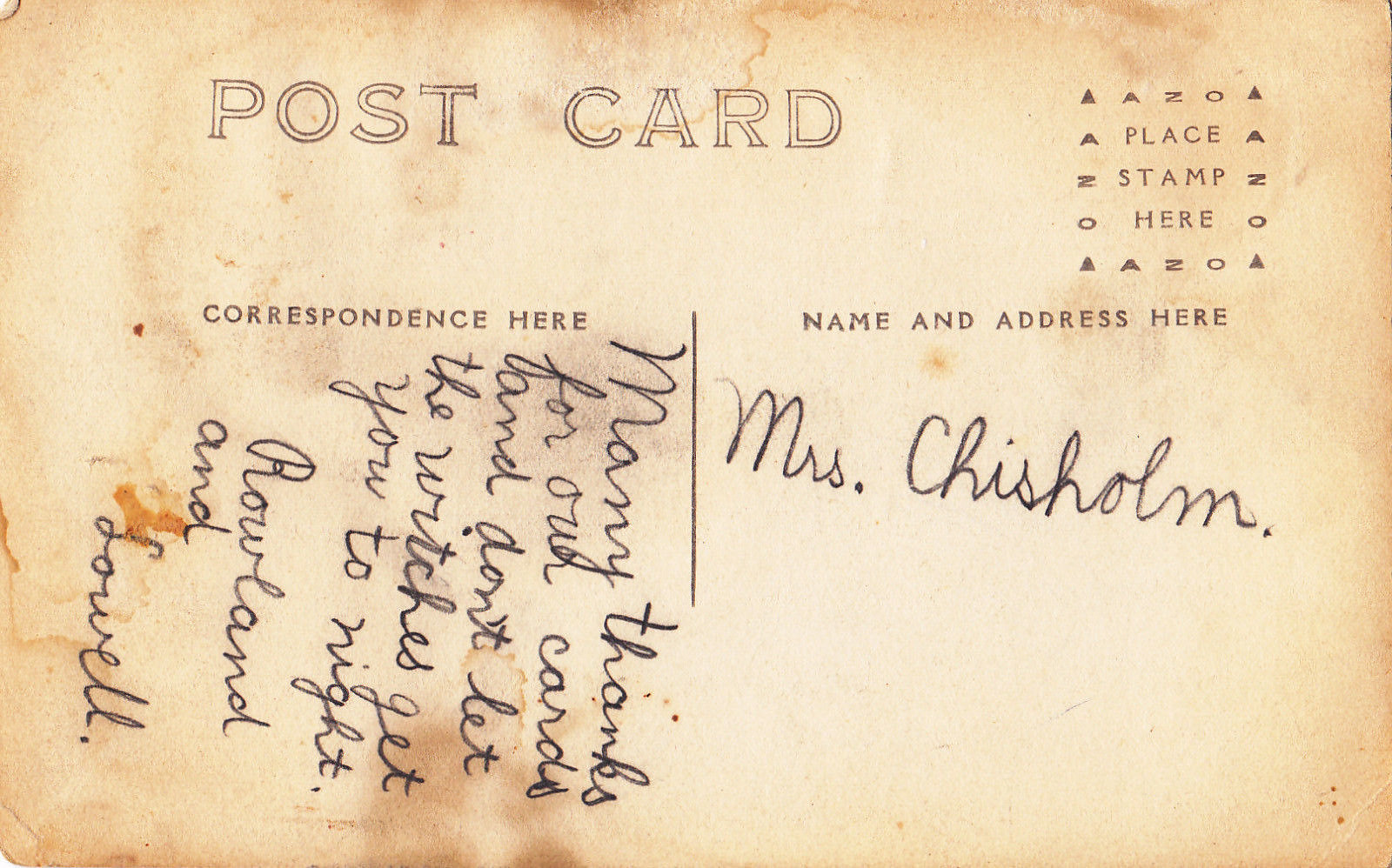This image shows the backside of a very vintage, outdated postcard characterized by its heavily discolored and worn paper that has taken on a brown and yellow hue. At the top, the word "POSTCARD" is printed in bold, black font. In the upper right corner, there's a designated area labeled "Place Stamp Here," although no stamp has been affixed. The postcard is divided into two sections by a vertical line: the left side is marked "Correspondence Here" and the right side "Name and Address Here."

Under the "Correspondence Here" section, a message written in black ink and cursive script reads, "Many thanks for our cards and don't let the witches get you tonight," signed by Roland and Laurel. On the right side, in the "Name and Address Here" section, the name "Mrs. Chisholm" is elegantly penned in upright cursive. The overall appearance of the postcard, with its yellowed and stained paper, reinforces its antiquated charm.